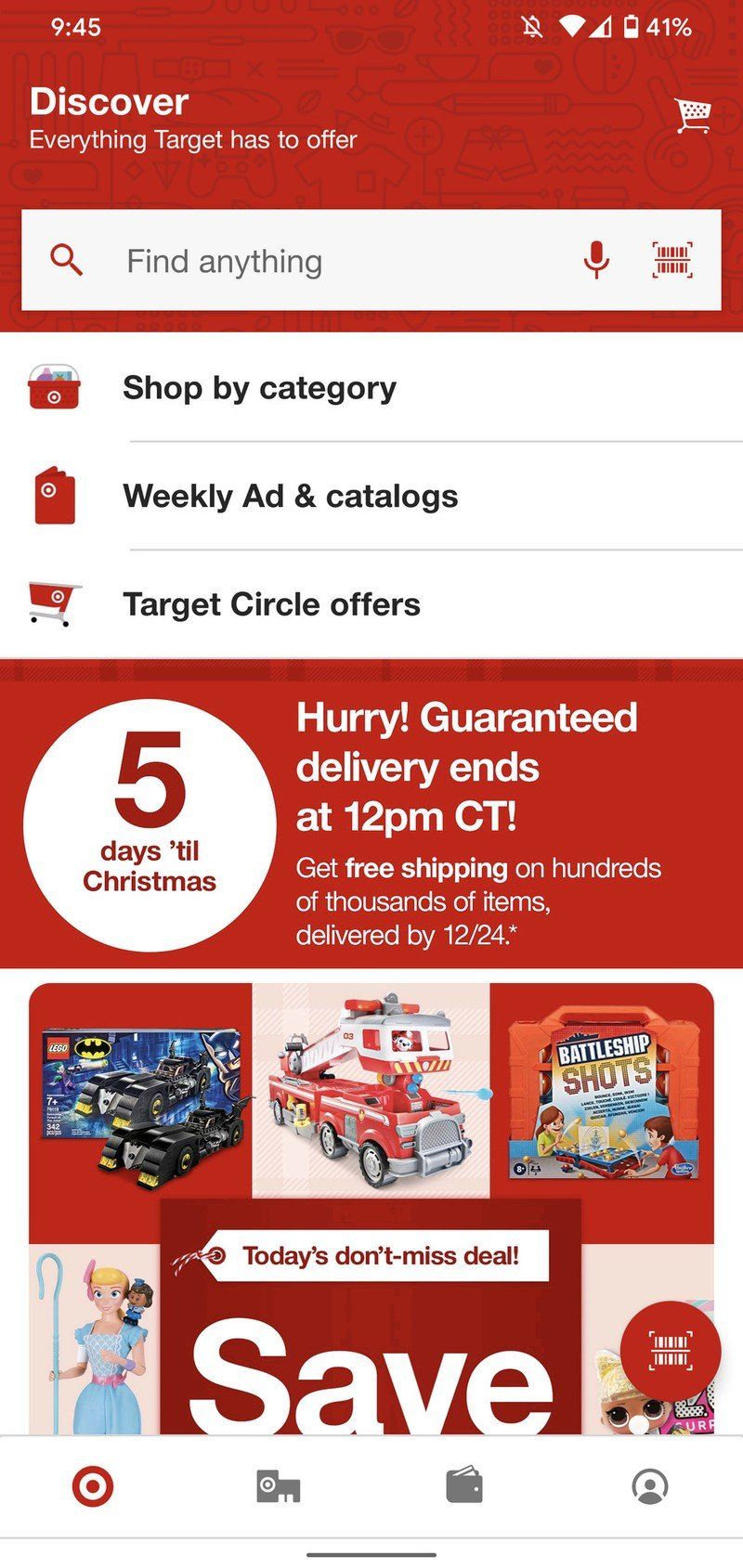The image, a vertical screenshot from a Target app or website, features a distinct red and white background. At the top left, the white text displays the time as 9:45. On the top right, white icons depict a bell, an upside-down triangle, and a battery indicator showing 41% charge. Below, in bold red text, is the word "Discover," with the phrase "everything Target has to offer" in less bold text beneath it. 

To the right is a shopping cart icon and a search box outlined in white, containing the prompt "Find anything." Next to this are icons for a microphone and a barcode scanner.

Further down, three black, bolded headings read "Shop by Category," "Weekly Ads and Catalogs," and "Circle Offers." Below is a red banner with a white circle, inside which red letters announce, "5 days till Christmas." Following this is the message in white, "Hurry! Guaranteed to arrive by 12 p.m. Central, get free shipping on hundreds of thousands of items, delivered by December 24th."

The bottom section displays images of various toys under "Today's Don't Miss Deal," accompanied by several icons at the footer.